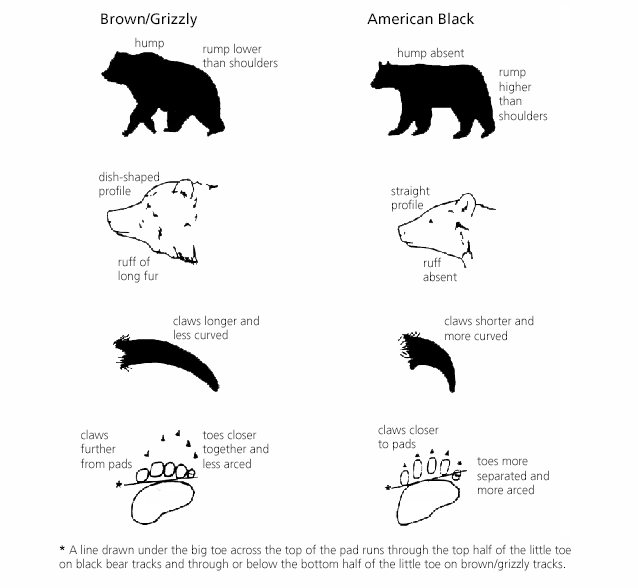This detailed poster is a comparative diagram highlighting the distinctions between brown (grizzly) bears and American black bears. The left side of the poster features the brown/grizzly bear, while the right focuses on the American black bear. Each side contains a series of four simplified illustrations with textual descriptions.

1. The first illustration is a side-view silhouette of the bears. The brown/grizzly bear silhouette has a notable hump just behind the head and shoulders, and its rump is positioned lower than its shoulders. Conversely, the American black bear silhouette displays no hump, with its rump higher than its shoulders.

2. The second illustration presents the profile of their heads. The brown/grizzly bear's head has a dish-shaped profile with a noticeable ruff of long fur extending from the back of the head to the shoulders. In contrast, the American black bear’s head exhibits a straight profile without the ruff of fur.

3. The third set of images shows the claws. The brown/grizzly bear claws are longer and less curved, compared to the shorter and more curved claws of the American black bear.

4. The fourth illustration depicts the paw prints of each bear. For the brown/grizzly bear, the claws are further from the pad, and the toes are closer together and less arched. The American black bear's paw print shows claws closer to the pad, with toes more separate and more arched.

An additional note at the bottom explains that for the American black bear's tracks, a line drawn under the big toe across the top of the pad runs through the top half of the little toe, whereas for the brown/grizzly bear's tracks, the line runs through or below the bottom half of the little toe. Each illustration is designed to be straightforward for easy understanding.